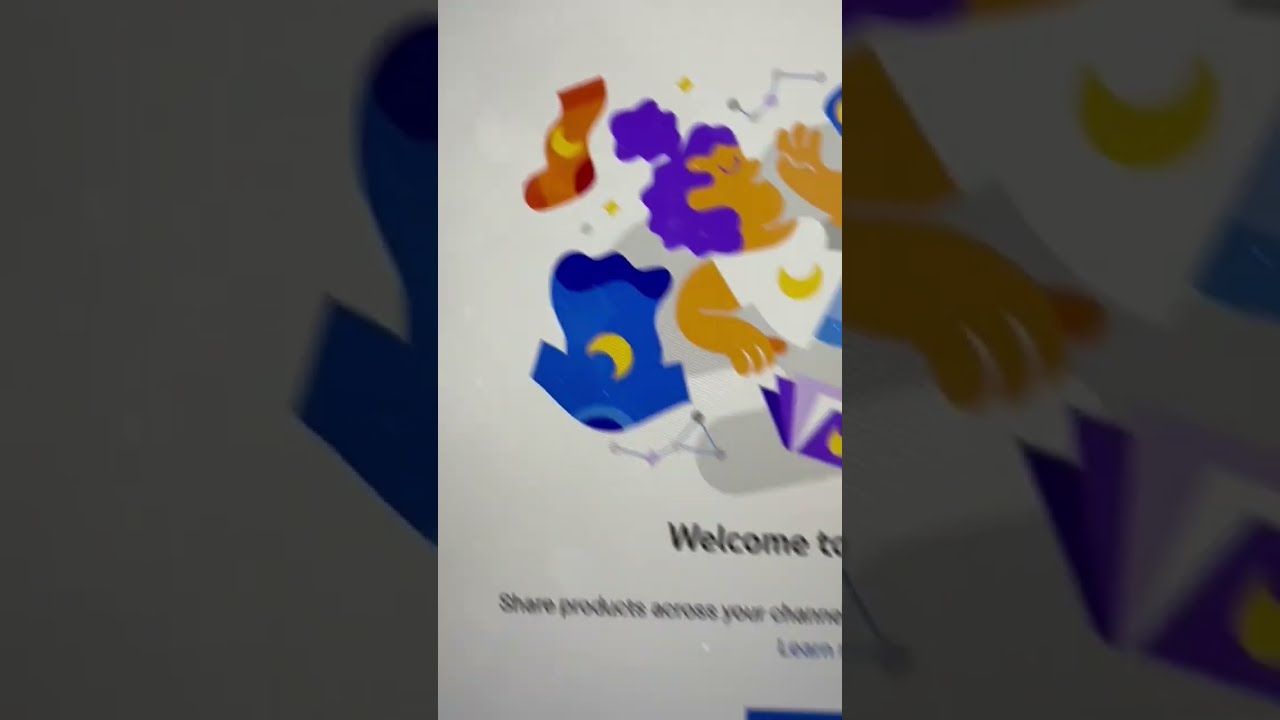The image depicts a blurry, cropped screenshot likely taken from a tablet or computer screen using a phone camera. In the center portion of the image against a white background, black font text says "Welcome to," followed by "share products across your channels," and a blue font button labeled "learn" below it. This text appears to be part of a sign-in or FAQ page designed to introduce users to a service, potentially a video streaming or product-sharing platform. Prominently, there is a colorful, cartoony illustration of a woman with orange-brown skin and purple hair, lounging back and appearing to sing. She wears a white t-shirt adorned with a yellow moon print. Surrounding her are various items of clothing and books featuring the same moon design, including a large blue t-shirt, brown socks, and several triangular constellation-like patterns. Darker side panels frame this central artwork, showing a partial outline of the blue t-shirt on the left and elements like an arm with hands and a moon with a purple triangle on the right.